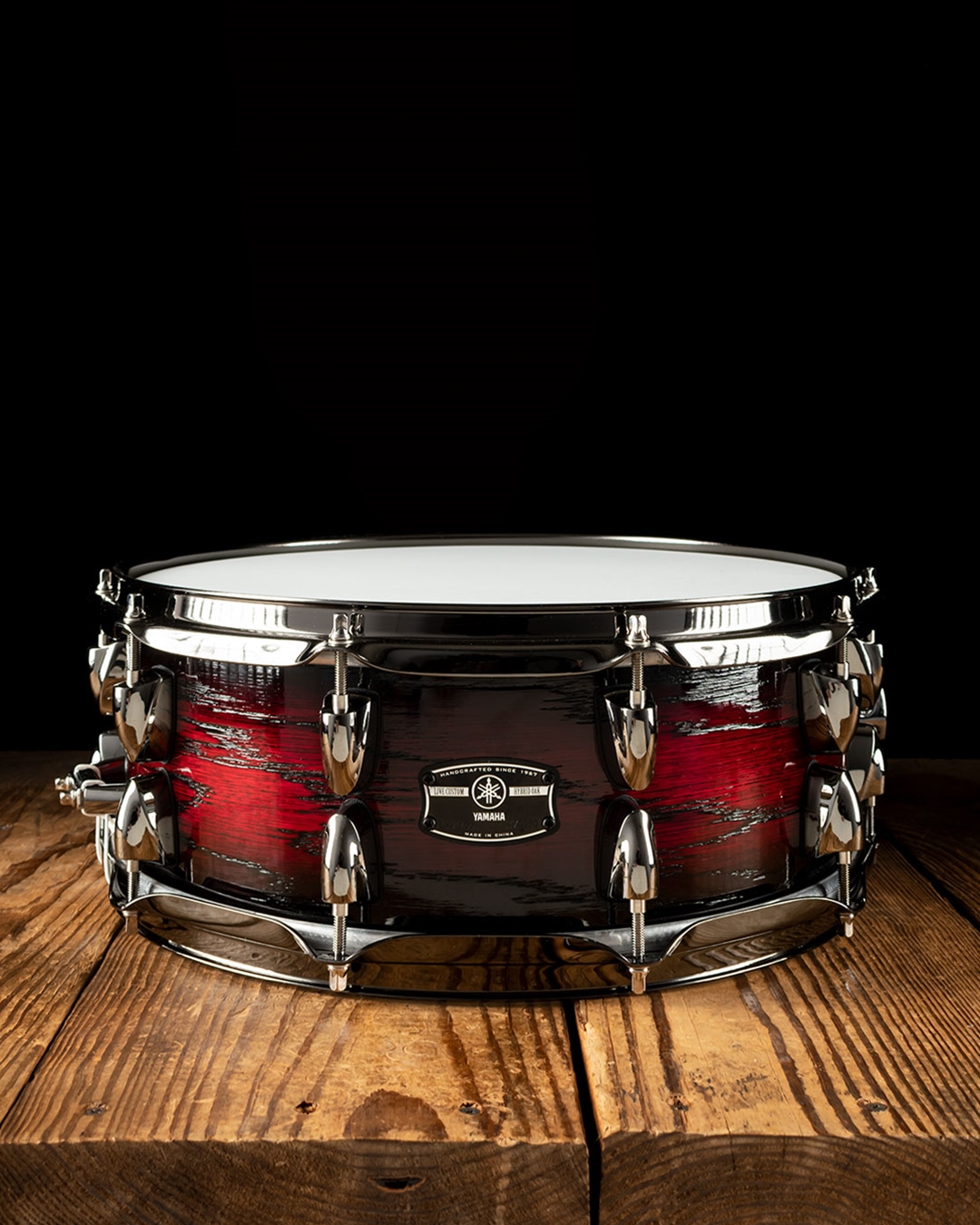The image features a vividly detailed, color photograph of a Yamaha snare drum resting on a rustic wooden table. The snare drum boasts a striking red shell with a deliberately worn, edgy appearance, accentuated by reflective chrome hardware. The drum's top striking surface is white, encircled by shiny silver rims, securely held by long silver screws. A black and silver logo plate with the word "Yamaha" and a distinctive six-pointed star is prominently displayed on the drum's front.

The table, constructed from thick, heavy, 2x4 wooden planks, exhibits a dark, grainy texture, possibly finished with varnish, and runs vertically across the image. The backdrop is entirely black, creating a stark contrast that highlights the drum's vibrant colors and metallic sheen. The light source adds a subtle shine, particularly on the top rim of the drum, giving it a polished and radiant appearance.